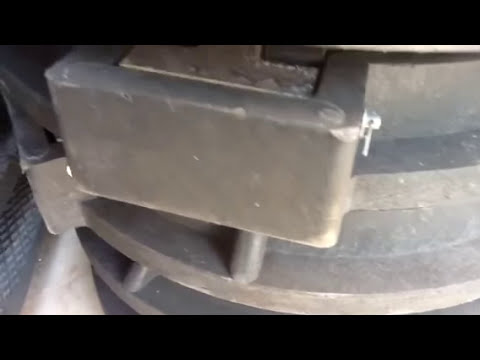The image shows a metallic device that appears intricate and somewhat obscured, making it difficult to identify its exact function. The device has a complex, mechanical structure featuring interconnected elements, suggesting it could be part of a larger machine or engine, potentially related to construction or automotive equipment.

At its center is a prominent rectangular steel structure that protrudes outward. Directly connected to this is a spherical component, indicating a possible pivoting or turnable function. On the left side of this central piece, there is a smaller rubber wheel, adding to the mechanical complexity. The entire assembly is characterized by additional ledges and edges, forming a multi-layered arrangement.

Further down, the object features a series of similar rectangular blocks, with the top one having a groove cut out that holds a barely visible attachment. One of these blocks is positioned higher on a circular section of the structure, while two others are situated below it, indicating a tiered design. The bottom-most level lacks these rectangular blocks entirely. On the side, there's a noticeable white lock secured with a pin.

The image is taken outdoors, and a metallic wall forms part of the background on the left side, contributing to the industrial and mechanical theme of the scene.